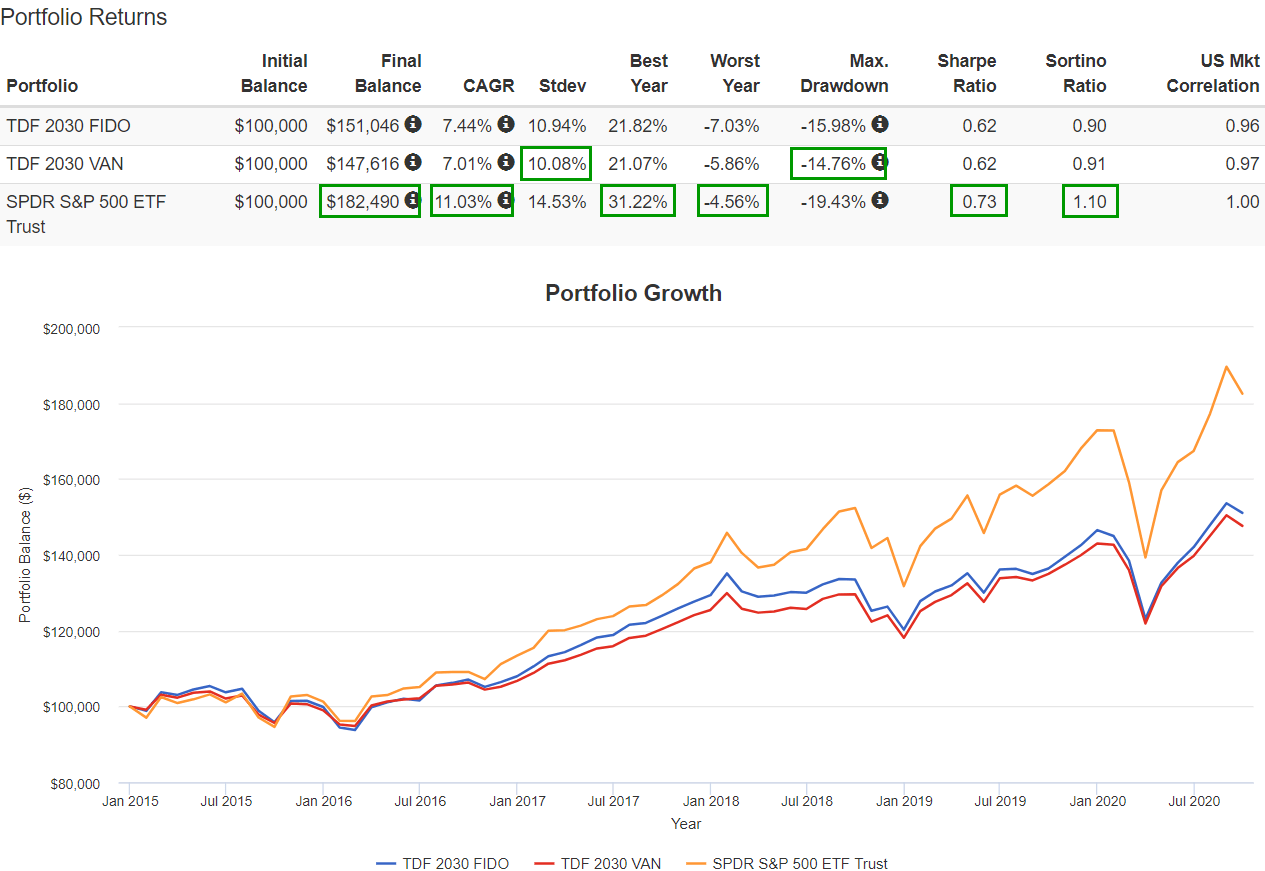A screenshot from Topsy's Portfolio Returns website displays three investment items: TDF 2030 Fido (F-I-D-O), TDF 2030 Van (V-A-N), and SPDR S&P 500 ETF Trust. The image includes a graph at the bottom that illustrates the growth trajectories of these three investments, all starting with an initial balance of $100,000. Notably, the SPDR S&P 500 ETF Trust exhibits the highest growth, reaching a value of $182,000, which approximates an annual growth rate of 11%.

Additionally, the screenshot contains various technical numbers and percentages, such as best and worst annual performances. The SPDR S&P 500 ETF Trust had a best year performance of a 31% gain and a worst year with a 4.5% loss. The image also displays the US market correlation coefficients for the investments, with the SPDR S&P 500 ETF Trust showing a perfect correlation of 1.00, while the TDF 2030 Fido and TDF 2030 Van have slightly lower correlations at 0.96 and 0.97, respectively.